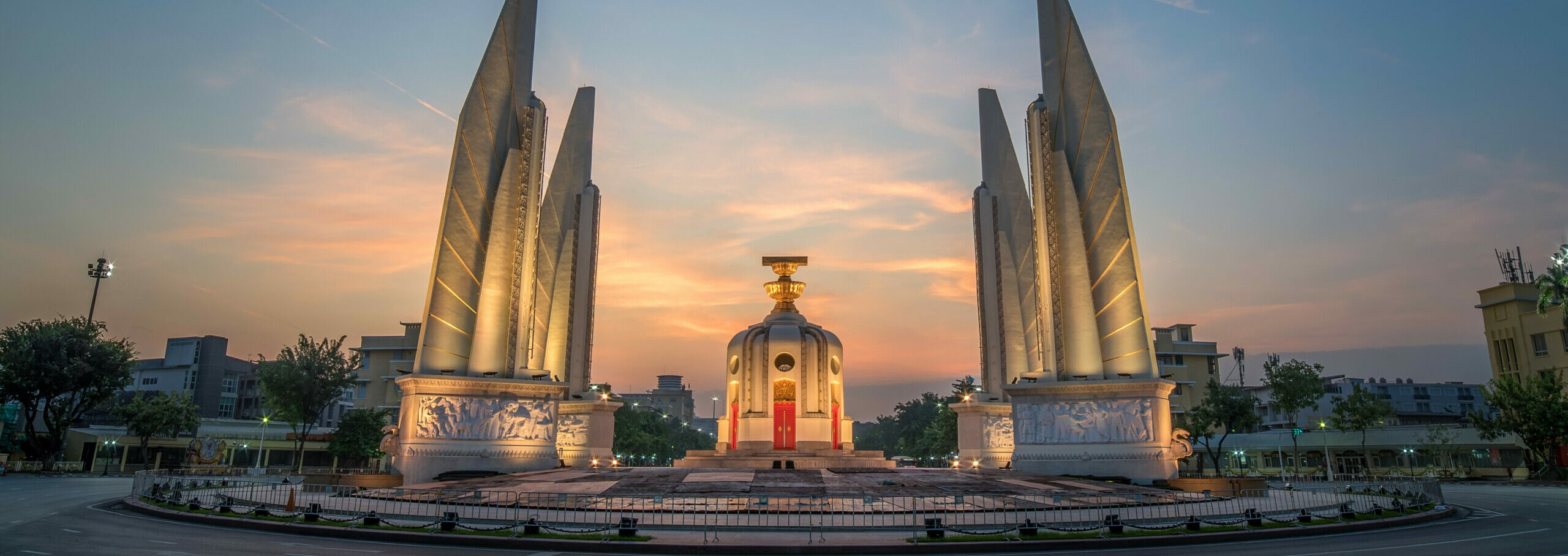The photograph displays a detailed and vibrant cityscape at dusk, featuring a grand central monument set against a backdrop of a mostly clear sky adorned with pink and orange clouds. At the heart of the image, the main monument is a circular cream-colored structure with red doors and a distinctive golden element at its top, resembling an inverted vase. Flanking this central structure, there are four tall, knife-like monuments with white bases and gray, blade-like structures accented with golden stripes, two on each side. These monuments and the central structure are enclosed by fencing, forming a circular arrangement in the middle of the scene. The surrounding area includes a mix of buildings, both tall and short, and green trees aligning a city street. Beyond this urban setting, the sea or ocean can be faintly discerned. The entire composition evokes a serene yet majestic urban environment, potentially within an unrecognized city.